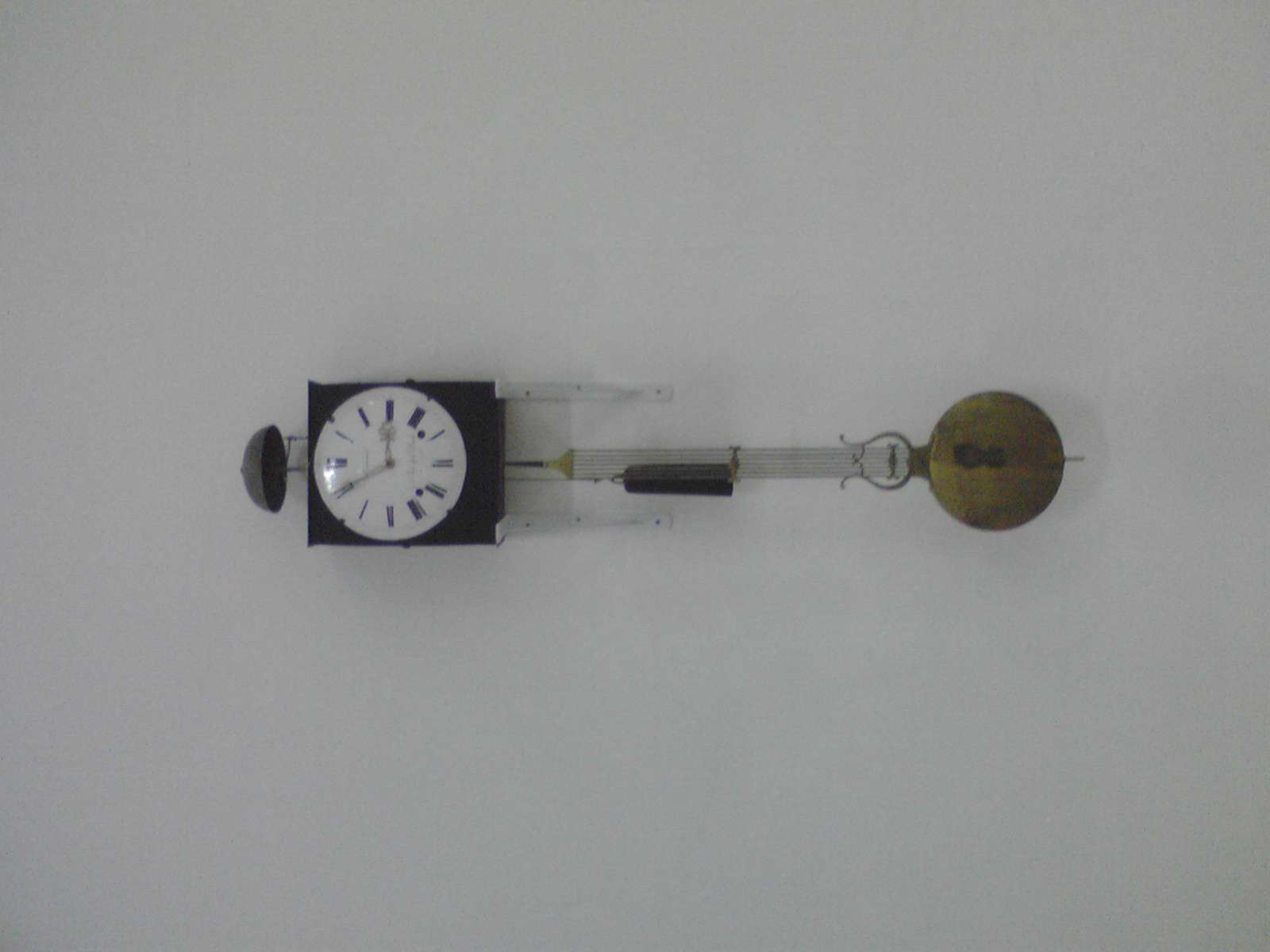This image features a horizontally oriented, real-life wall clock, giving it an abstract appearance. The clock is square-shaped with a black border and a circular white face. The hour markers are represented by varying thicknesses of stripes rather than traditional numbers, and the hands of the clock possess an antique, ornate design, possibly in a golden or bronze hue. At the top of the clock, there is a smaller cap that resembles the top of an old bell, patinaed to a darker gray. Extending from this cap is an elaborate, bronze, ornate piece that includes thin wires or string-like elements. Attached to the end of these strings is a large, round, bronze pendulum with small black dots, contributing to the clock's abstract and artistic quality. The clock is set against a medium gray background, further highlighting its unique and unconventional presentation.